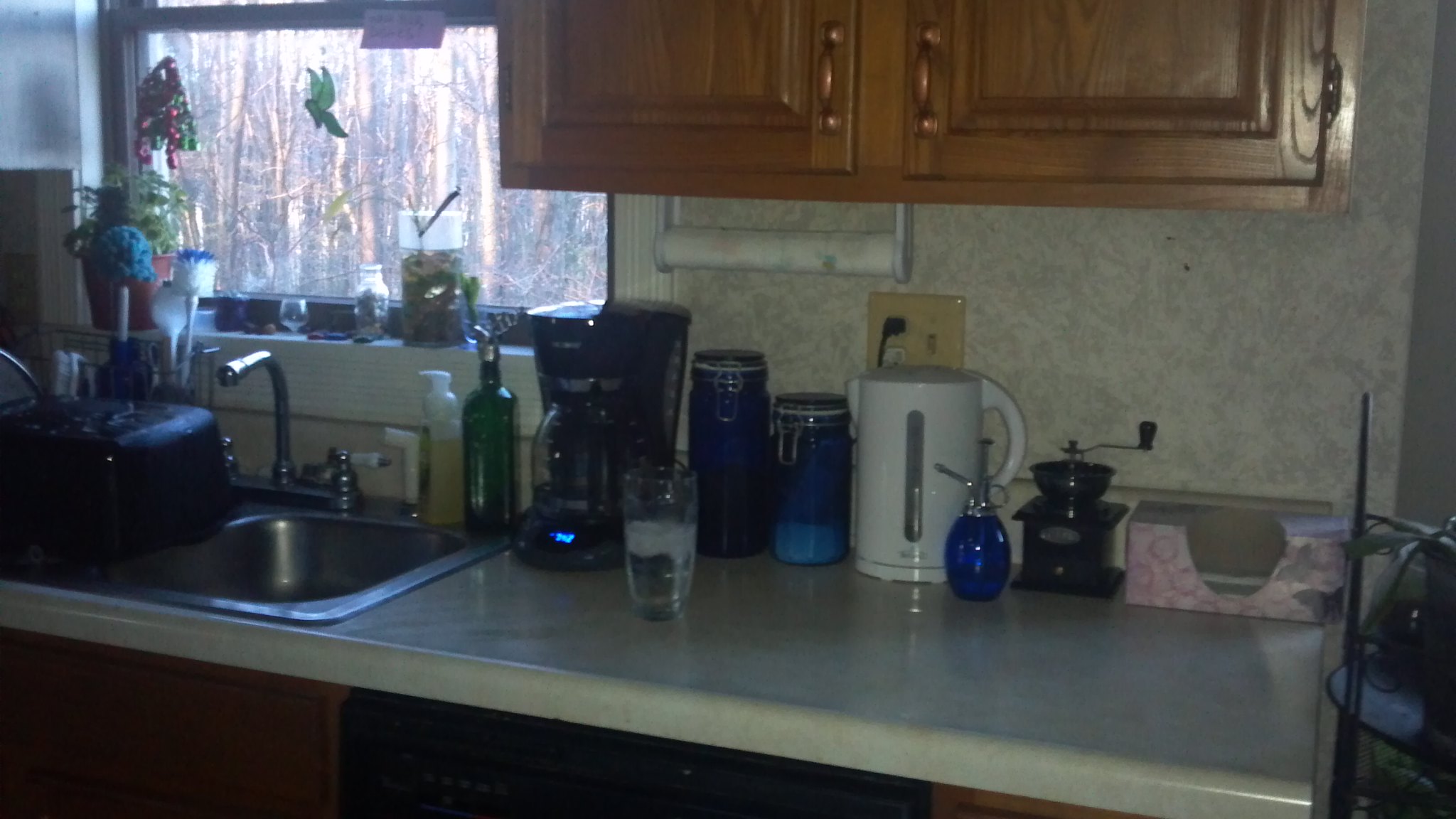This color photograph, slightly out of focus and taken in landscape orientation, depicts an older kitchen counter with a white Formica surface and a distinctive drip edge. The counter, sloping from bottom right to middle left, is cluttered with various kitchen items, including a blender, a coffee maker, a vintage coffee grinder, a half-full glass of iced water, and a mostly empty box of pink tissues. There are also two blue glass jars, a green glass bottle of olive oil, a hot water kettle, and a green glass plant mister. 

Central to the image is a double stainless steel sink with a high-arched faucet featuring porcelain grips, sitting below a wooden wall cabinet equipped with brass-colored handles. The almost empty paper towel roll holder attached beneath this cabinet emphasizes the kitchen's well-used, lived-in feel. Above the sink is a window through which trees are visible, allowing natural light to filter into the somewhat dim scene. The windowsill is adorned with planter-type clear jars, glass vases, and a potted plant, with a distinctive sun catcher in the shape of a green bird hanging centrally. The window itself has a see-through design stuck to the glass, adding to the visual complexity of the image.